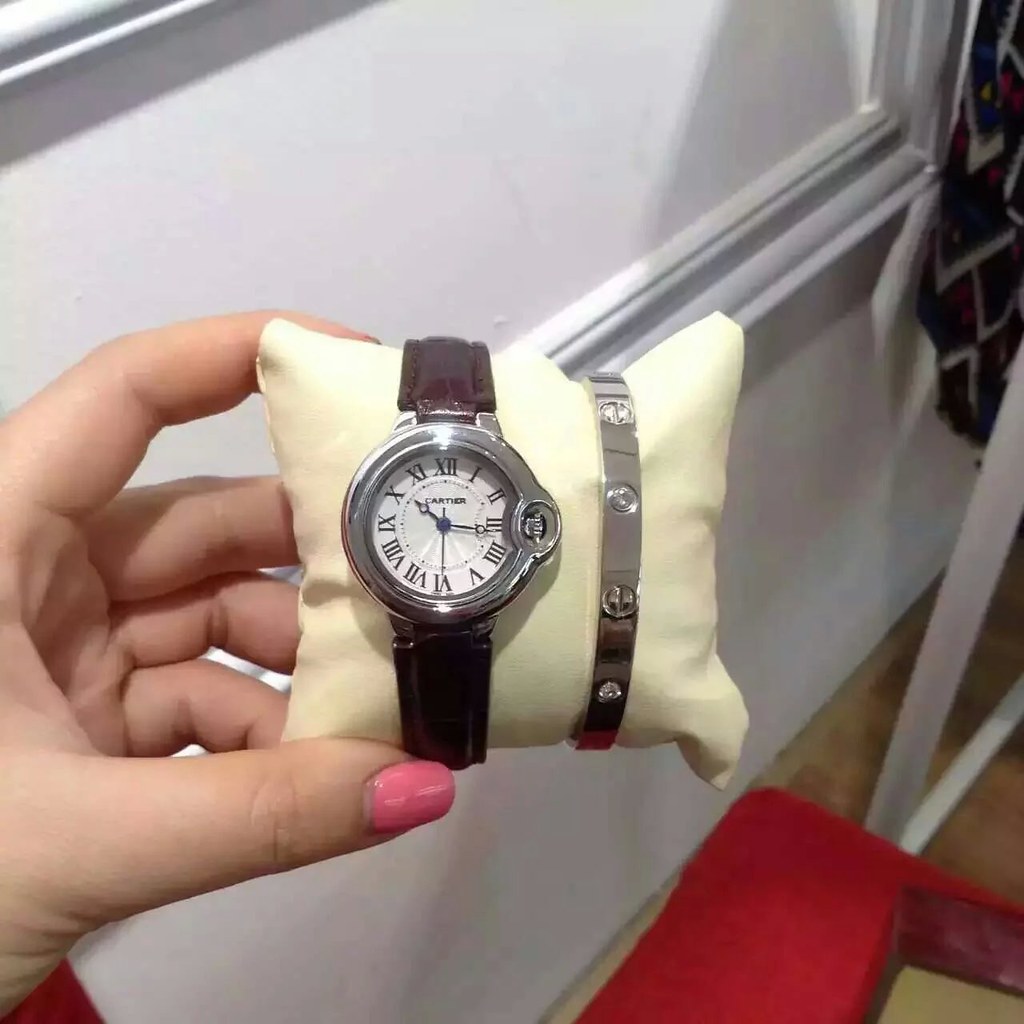In the photograph, a woman's left hand, adorned with pink nail polish, delicately holds up a small yellow pillow. Resting on the pillow are a Cartier watch and a Cartier bracelet. The watch features a brown leather strap and has a distinctive Cartier face, complete with Roman numerals and a potential stone on the stem where the time is set. Surrounding the face is a casing that appears to be either white gold or sterling silver. Beside the watch, the bracelet is also recognizable as a Cartier piece, adorned with the brand's iconic round screws, suggestive of a design that might need a screwdriver and composed of interconnected white gold links. The background reveals a wooden floor, with a hint of something red and white beneath, possibly a cushion, table, or fabric, adding an additional layer of texture to the scene. The photo's depth and artificial lighting suggest the time captured may be around 10:15 PM.